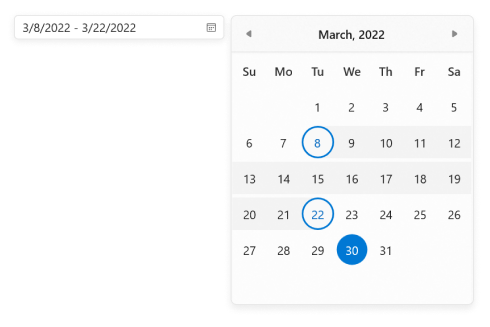The image features a predominantly white background. On the left side, there is a text box displaying the date range "3/8/2022 through 3/22/2022." Adjacent to this text box, towards the right, is a search bar containing a calendar icon. 

To the right of the search bar, a calendar for March 2022 is displayed. At the top of the calendar, there is a left-facing arrow and a right-facing arrow, enabling navigation between months. The days of the week are labeled in a row across the top: Sunday, Monday, Tuesday, Wednesday, Thursday, Friday, and Saturday.

The first day of the month lands on a Tuesday, thus the days are arranged in numerical order, starting from Tuesday the 1st and ending with Thursday the 31st. The numbers are against a light gray background. 

Significant dates stand out with special formatting:
- The 8th of March, a Tuesday, is marked with blue text and encircled by a blue ring.
- From the 9th to the 21st of March, the dates are in a darker font with a contrasting darker gray background.
- The 22nd of March, also a Tuesday, is similarly highlighted with blue text and a blue circle around it.
- The 30th of March is distinctly highlighted with a solid blue circle, and the number inside it is in white or a very light gray text.
- The 31st of March returns to the standard format, with no special markings.